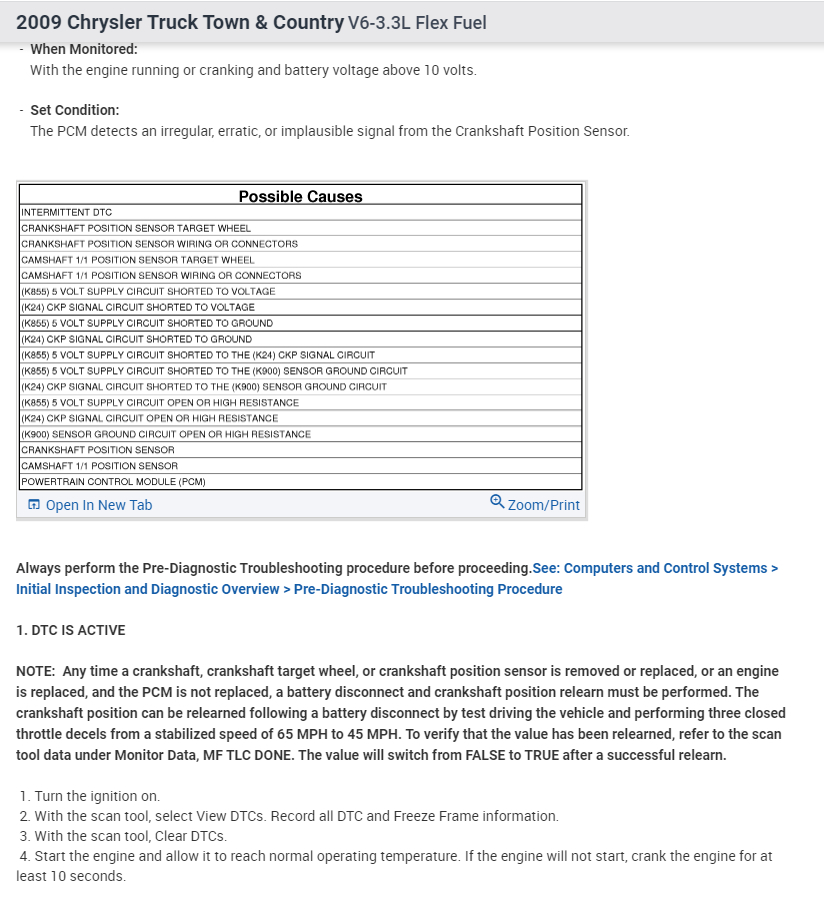The image depicts a comprehensive troubleshooting guide specifically for the crankshaft position sensor of a 2009 Chrysler Town & Country V6 3.3 liter flex-fuel truck. The guide focuses on identifying potential issues that may cause the Powertrain Control Module (PCM) to detect irregular signals from the crankshaft position sensor. Highlighted potential causes include problems with the sensor's wiring, connectors, and circuits.

The guide advises technicians to examine Diagnostic Trouble Codes (DTC) and undertake necessary repairs. It also outlines the steps needed to relearn the crankshaft position sensor if related components are replaced. The importance of always performing the pre-diagnostic troubleshooting procedure before any further action is stressed to avoid potential dangers.

The document notes that when monitored, the engine must be running or cranking with a battery voltage above 10 volts. In cases where the PCM detects an erratic or impossible signal from the crankshaft position sensor, the guide lists approximately 12 potential causes. The details underscore the complexity of diagnosis and repair for this component, emphasizing the intricacies and challenges involved in the troubleshooting process.